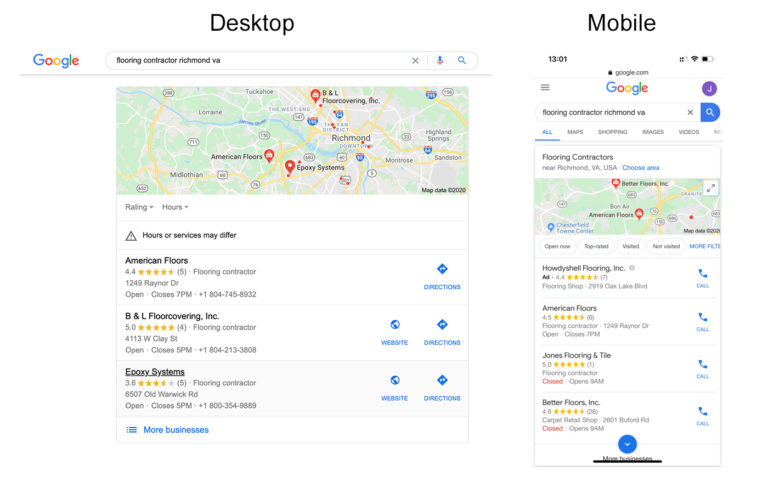The image depicts a comparative study of search results for "flooring contractor Richmond VA" conducted on Google from a desktop computer (on the left) and a mobile device (on the right). The search results, although initiated using identical keywords, display notable differences in their order and entries.

On the desktop version, the top three results are "American Floors," followed by "B&L Floor Covering Incorporated," and then "Epoxy Systems." Contrarily, the mobile search provides "Howdy Shell Flooring Incorporated" as the first result, then "American Floors"—the only common listing with the desktop search—and the third and fourth results are "Jones Flooring and Tile" and "Better Floors Incorporated," respectively.

Additionally, both platforms show a map displaying the locations of the flooring contractors. The desktop version's map is substantially larger, showcasing all three top flooring sites prominently marked. In contrast, the mobile version's map is significantly smaller—approximately a quarter of the desktop map's size—and displays only two of the flooring stores.

This intriguing comparison highlights the differences in search result algorithms and display formats between desktop and mobile devices.